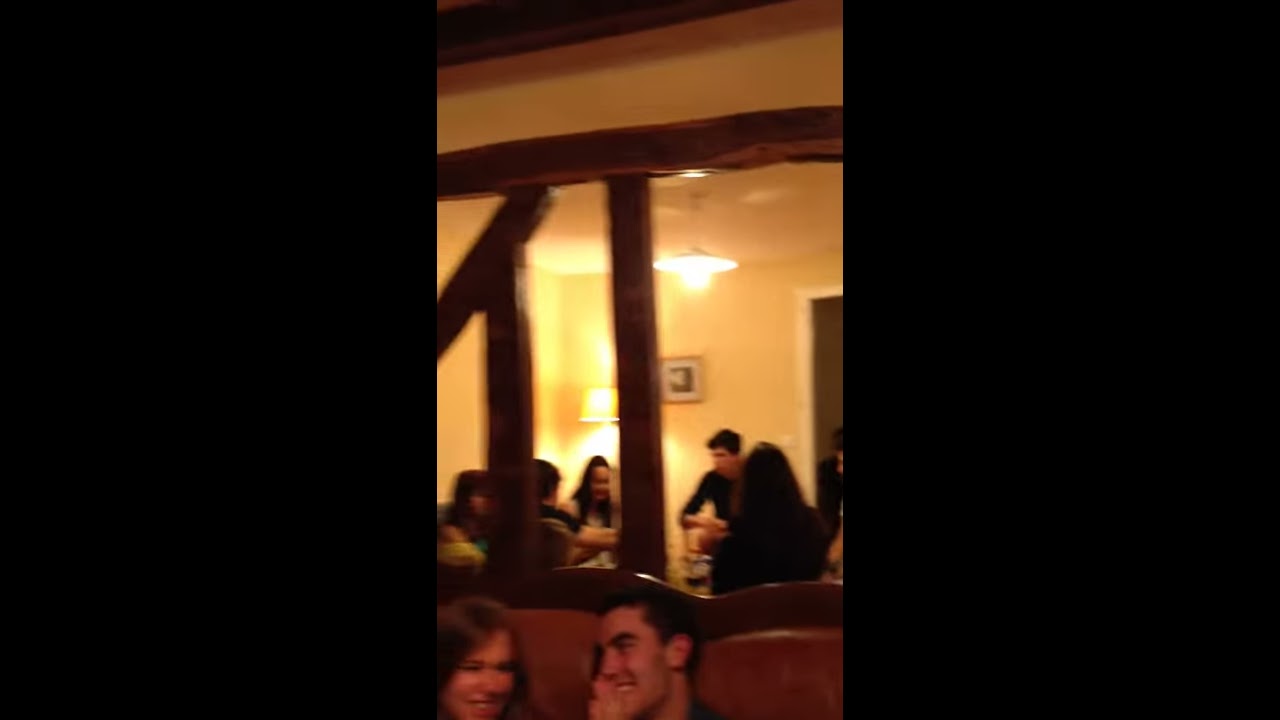The image is a blurry, dimly-lit photograph from a gathering, likely a party, with a cozy, intimate atmosphere. In the immediate foreground, there's a couch with red cushions featuring two young white people, a man and a woman in their twenties, their heads close together, sharing a laugh. The man, with short black hair, is seated centrally and looks to his left at the woman, who has long brunette hair. Only their faces are visible as the photo is tightly cropped at the bottom.

Behind them, partially obscured by wooden support beams, another room is visible. Here, a group of young people, all engaged and seemingly enjoying the moment, are gathered around a table or in a circle. The background shows yellow walls and a sliding glass door partly cropped to the right. A lamp and a ceiling lighting fixture illuminate the scene, hinting at a homey setting. Among the party-goers, one man is holding a guitar, suggesting a musical element to the gathering. The entire scene, captured possibly on a shaky camera phone, exudes warmth and camaraderie despite the blur.